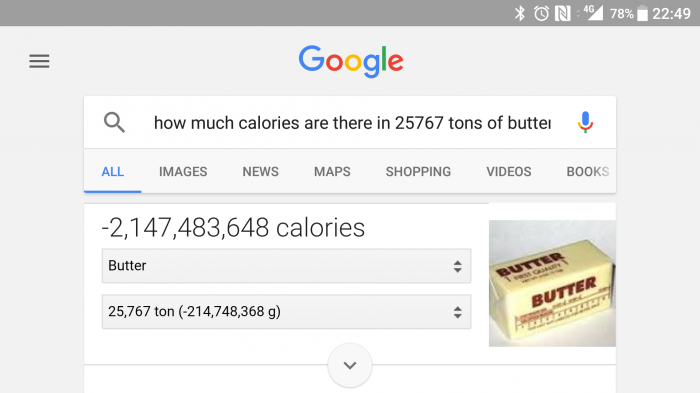A screenshot of a Google search on a smartphone is displayed. The status bar at the top shows a 4G connection, a 78% battery level, and the time as 22:49. The Google logo appears in its traditional colors: blue, red, yellow, and green, situated above a large search bar. Inside the search bar, the query reads, "how much calories are there in 25,767 tons of butter" in lowercase black letters, accompanied by a blue microphone icon on the right.

Below the search bar, tabs for "All" (highlighted in blue and underlined), "Images," "News," "Maps," "Shopping," "Videos," and "Books" are visible. The primary search result under the "All" tab indicates a negative figure: "-2,147,483,648 calories." Directly underneath this, the word "butter" appears with an arrow that provides options to navigate up or down through results. Beneath that, the conversion of 25,767 tons into grams is shown in parentheses as "(negative 214,248,368 G)." On the right side of this conversion, there is an image of butter packaged in a container.